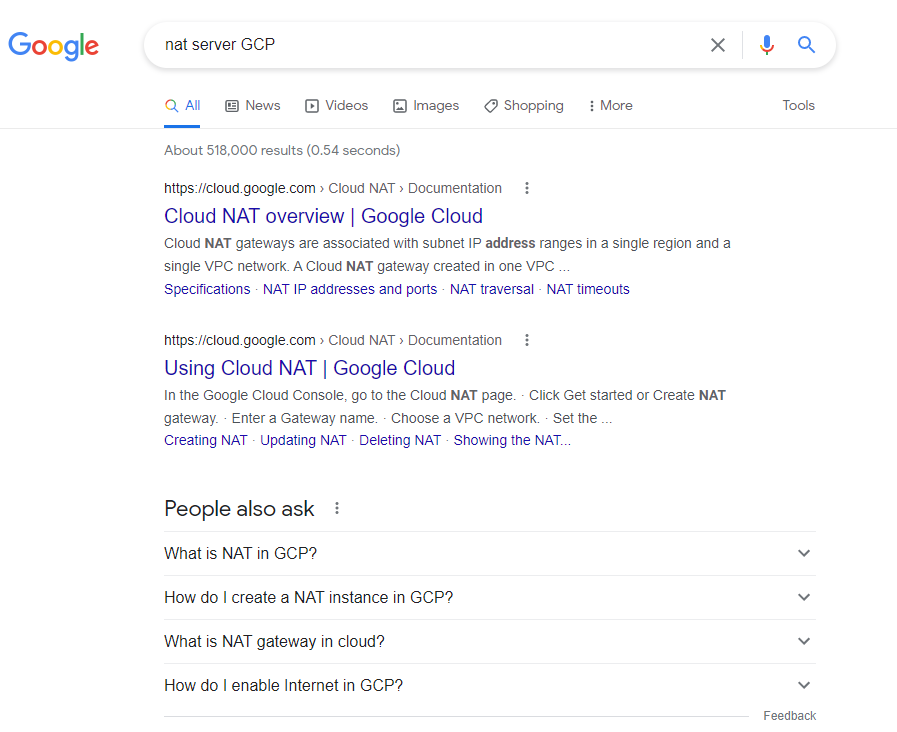This screenshot captures a Google search interface. In the top left corner, the iconic Google logo is displayed in its signature blue, red, yellow, and green color scheme. Adjacent to the logo is the search bar, which contains the query "NatServerGCP." Below the search bar, there are various section tabs, including "All," "News," "Videos," "Images," "Shopping," and a "More" option. To the far right, we see the "Tools" button.

The displayed search results include two primary links. The first result is from https://cloud.google.com, titled "Cloud NAT Overview," and the second, also from google.com, is "Using Cloud NAT." Beneath these two results is the "People Also Ask" section, featuring four expandable questions: "What is NAT in GCP?", "How do I create a NAT instance in GCP?", "What is NAT Gateway in Cloud?", and "How do I enable internet in GCP?" At the very bottom of the screenshot, there is a "Feedback" hyperlink, inviting users to provide feedback on the search results.